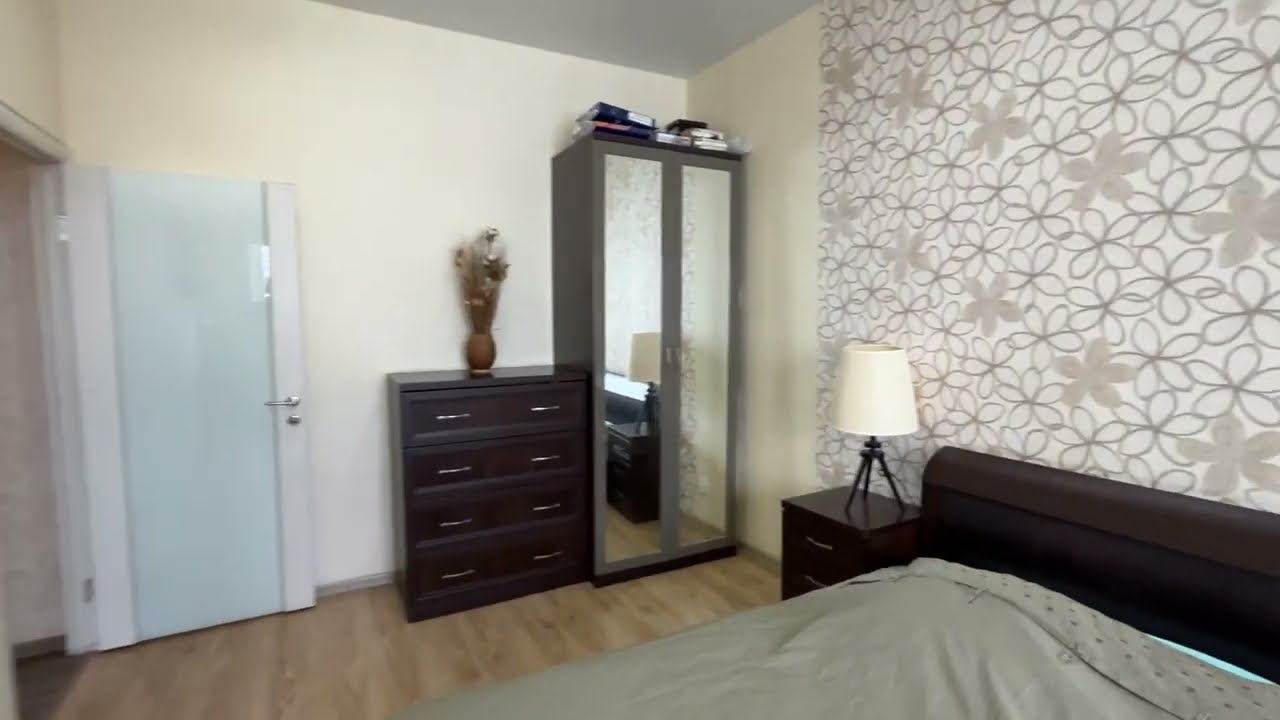This photograph captures a detailed view of a bedroom. On the left side, there's a partially open door with light blue and white panels, featuring a silver handle and frosted glass. The walls are painted a cream color, with the exception of the wall behind the bed, which is adorned with a white and tan floral print wallpaper. A wooden cabinet sits against the front wall, accompanied by a dark brown chest of drawers that holds a vase filled with artificial flowers. Adjacent to this, a tall, mirrored metallic wardrobe stands, with some files placed on top.

The floor is light brown wood with various shades, partially obscured by a bed. The bed has a dark brown leather headboard and is dressed with a gray bedspread and light blue sheets. A brown wooden bedside table is positioned next to the bed, topped with a white shade lamp that has dark tripod legs.

Overall, the room feels warm and coordinated with its brown, cream, and light blue color palette, augmented by floral accents and mirrored surfaces that add a touch of elegance to the cozy space.